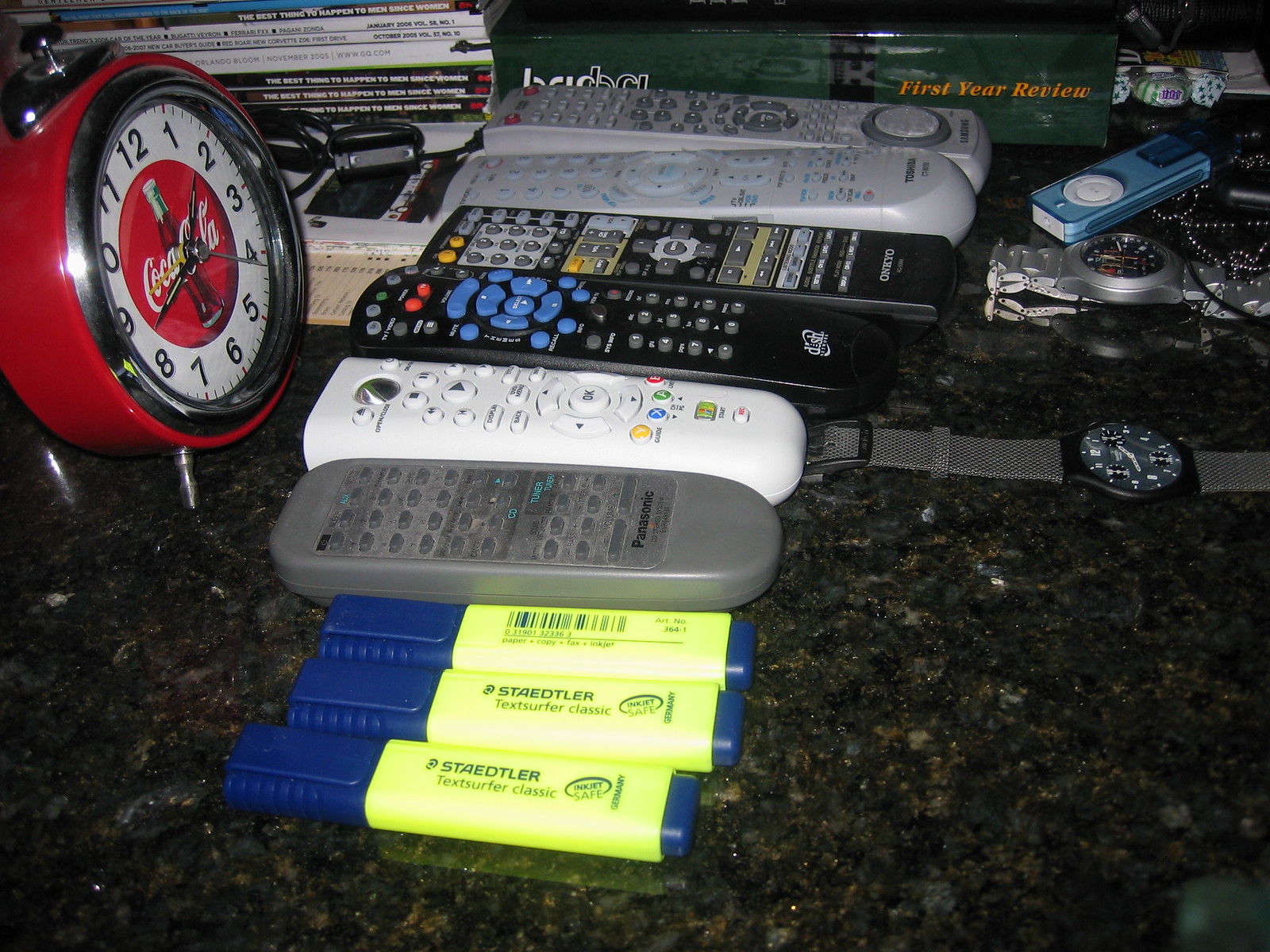In this landscape-oriented image, a variety of items are neatly arranged on a countertop, potentially set up for sale. Dominating the scene are six remote controls from different brands: a gray Panasonic remote, remotes for Dish Network, ONKYO, Toshiba, and Samsung, as well as an unbranded white remote. Elsewhere on the countertop are three yellow Staedtler highlighters with blue caps, an iPod Nano, a couple of watches, an assortment of books and magazines, including what seems to be either Maxim or Playboy, and a retro-style Coca-Cola alarm clock with a red rim, white face, black hands, and a red circle in the center displaying the Coca-Cola logo.